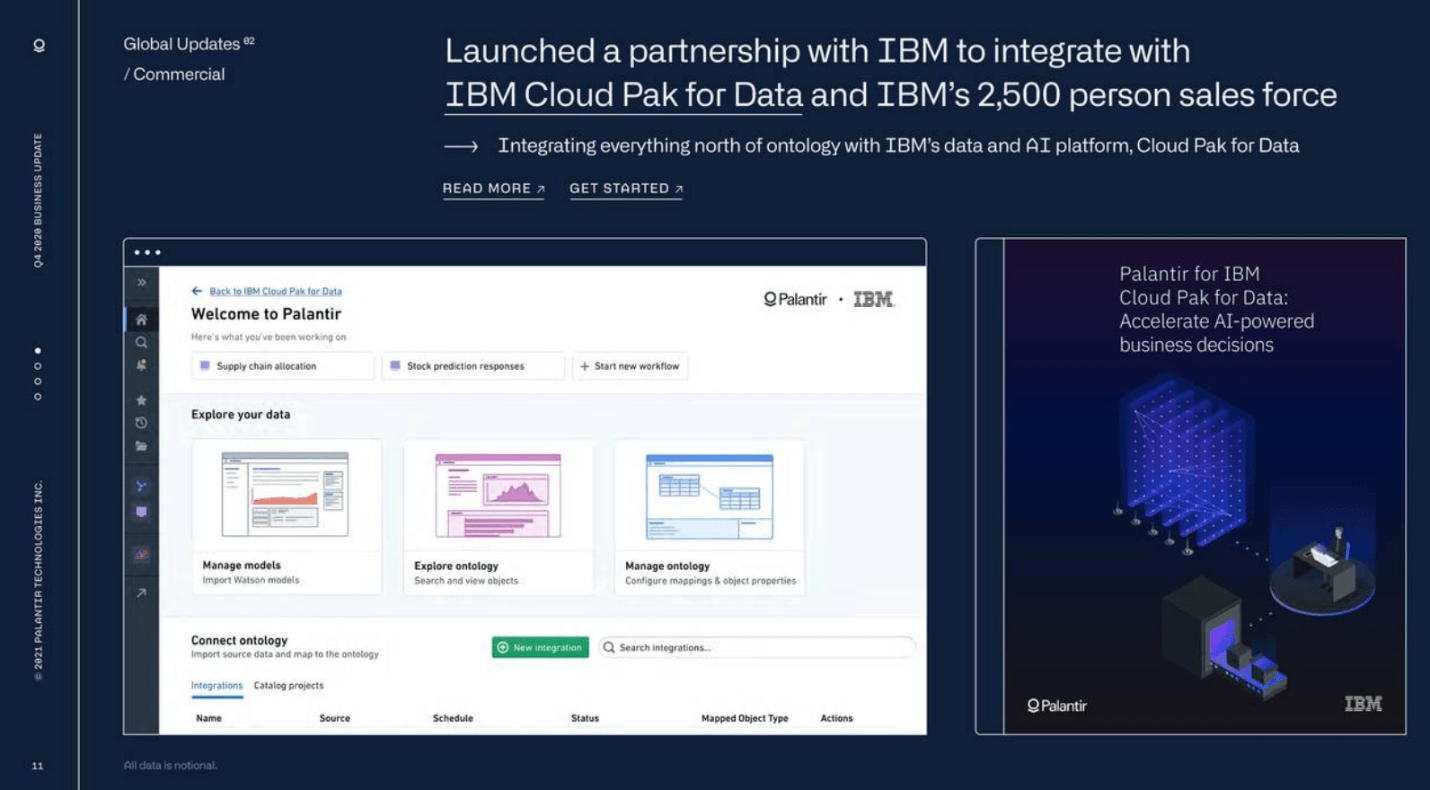The image captures a promotional announcement for a collaboration between IBM and Palantir. The title prominently reads, "Welcome to Palantir: Explore Your Data." Below, it highlights, "Global Updates / Commercial," suggesting the announcement is of significant global and commercial relevance.

The header indicates the launch of a partnership with IBM to integrate Palantir's capabilities with IBM's Cloud Pak for Data, a comprehensive data and AI platform. The text further elaborates that this integration involves IBM's 2,500-person sales force, aiming to streamline and enhance their data and AI efforts above a certain operational threshold.

Central to the image is the tagline, "Palantir for IBM Cloud Pak for Data: Accelerate AI-Powered Business Decisions." The graphic design includes an illustration of a person seated at a desk, working on a computer. The computer is depicted emitting a series of dots and lights, symbolizing data and connectivity. This visual flow transitions into a factory scene, emphasizing the end-to-end data ecosystem from analysis to tangible product output.

Overall, the detailed depiction underscores the strategic alliance between Palantir and IBM, highlighting the integration of advanced data analytics and AI to drive business innovation and efficiency.